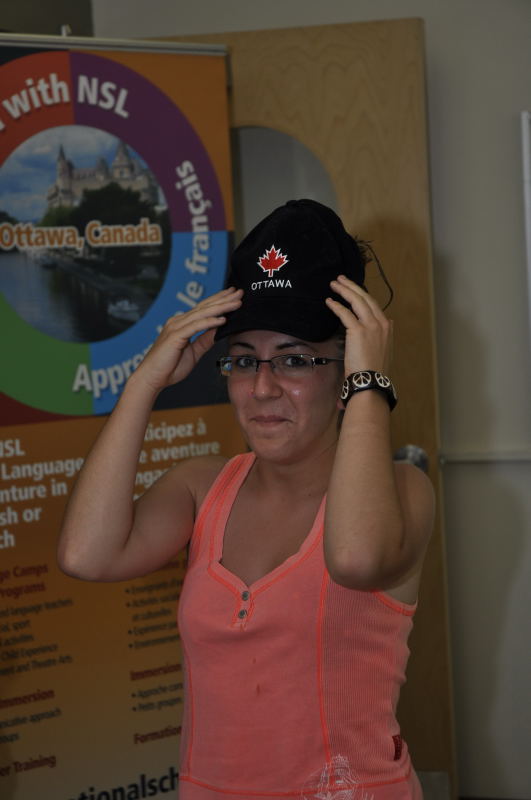The image features a woman with her hands raised, holding a black hat with a red Canadian maple leaf and the word "Ottawa" written on it just above her head. She is wearing glasses and a peach-colored tank top with two buttons at the front. On her left wrist, she sports a black bracelet adorned with silver peace signs. The setting appears to be indoors with dark, poor lighting. Behind her, there's a prominent banner with multiple colors, including red, purple, blue, green, and orange. The banner displays text in both English and French, including phrases like "NSL Ottawa Canada" and "Le Francais." Additionally, the background features a brown door and gray walls, adding to the indoor ambiance. She is looking directly at the camera with a slight smile, and the photo captures her from the waist up.